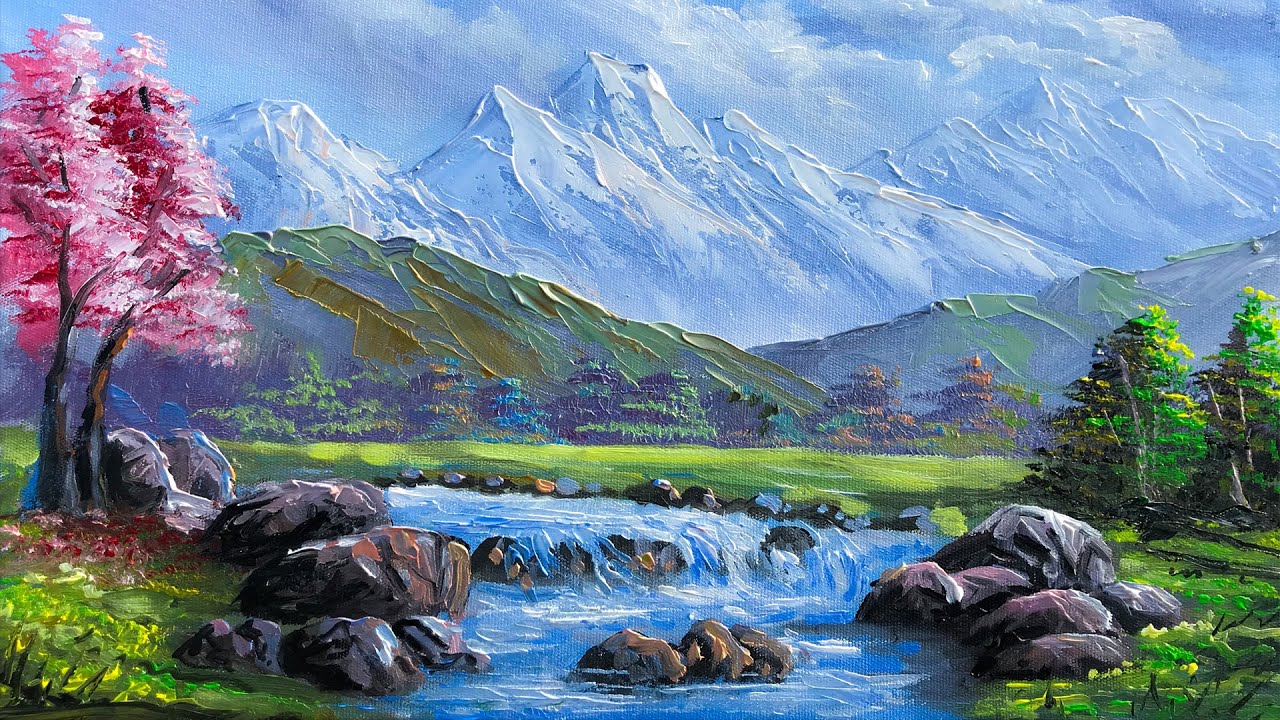This painting captures a serene and picturesque outdoor scene, emphasizing nature's beauty through a blend of vibrant colors and textured elements. The sky is a mix of blue and white, scattered with clouds, creating a peaceful backdrop. Dominating the distant background are tall, snow-capped mountains flanked by smaller, green hills. At the forefront, on the left side, stands a prominent cherry blossom tree with striking pink leaves, adding a pop of color. Below the mountains, the terrain transitions into grassy hills dotted with trees and rocks. A lively stream or creek cuts through the middle of the image, its flow interspersed with boulders, enhancing the scene’s idyllic quality. Alongside the stream, patches of flowers in yellow and maroon add further detail, while the plant life, including deciduous trees and vibrant foliage in blues, greens, and oranges, enriches the overall wilderness and nature theme of the artwork.